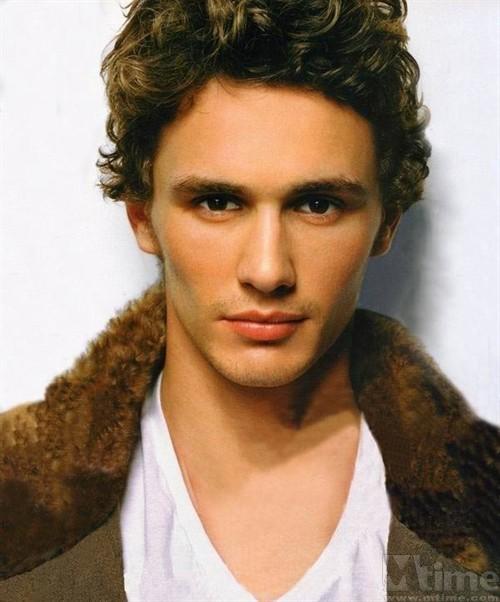The close-up photograph showcases a younger man, possibly James Franco, against a white backdrop. His hair is brown, wavy, and somewhat unruly, giving a messy yet intentional look. He has a light five o'clock shadow and a square jawline, exuding a confident and self-assured demeanor. He is wearing a white v-neck t-shirt beneath a distinctive jacket featuring a thick, brown, furry collar that arches behind his neck and slopes down over his shoulders. The image is cropped above his head and at chest level, making the top of his hair and lower body difficult to discern. A slight grayish shadow is cast on the wall behind him. In the lower right-hand corner, the text "m-time.com" appears partially transparent, suggesting it might be an advertisement or related content. The overall impression is of a stylish and conventionally attractive young man, likely in a modeling context.